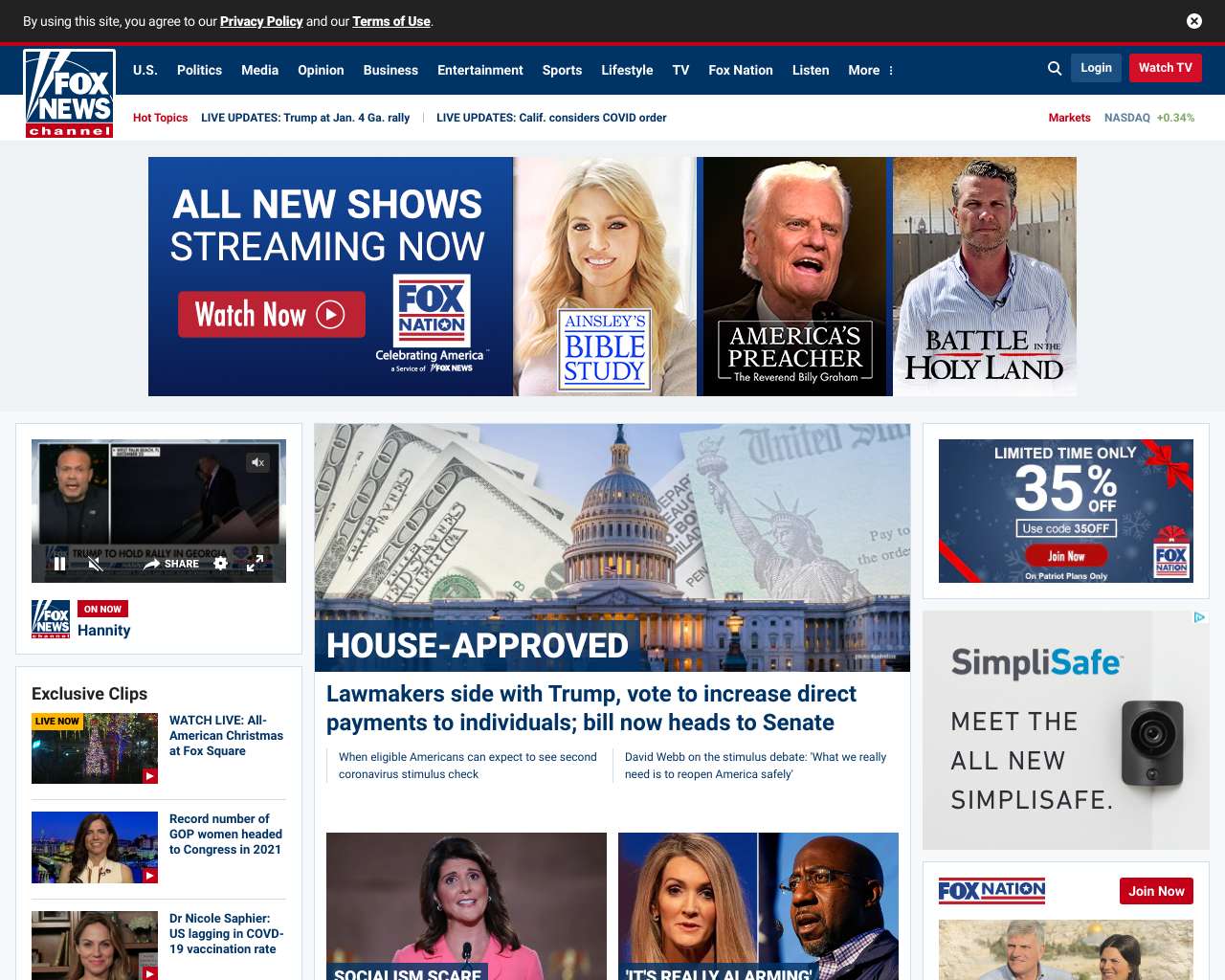Here is the cleaned-up and detailed caption for the described image:

---

The image depicts a slightly horizontally rectangular view of the Fox News Channel website's homepage. At the top of the page, next to the right of the prominent Fox News Channel logo, is a narrow horizontal blue banner featuring navigation options labelled: U.S., Politics, Media, Opinion, Business, Entertainment, Sports, Lifestyle, TV, Fox Nation, Listen, and More. On the far right of this blue banner are icons for search, login, and watch TV.

Directly below this banner is a larger rectangular horizontal advertisement announcing "All New Shows Streaming Now," accompanied by a "Watch Now" button, and the Fox Nation logo situated to its right. Adjacent to the advertisement are promotional images and titles for three featured shows: "Ainsley's Bible Study," "America's Preacher: The Reverend Billy Graham," and "Battle in the Holy Land."

Beneath the promotional content, the webpage is divided into three vertical columns. The central column is the widest, flanked by two narrower columns on each side. These columns contain a variety of news stories and articles. The rightmost column also features a couple of advertisements interspersed among the articles.

---